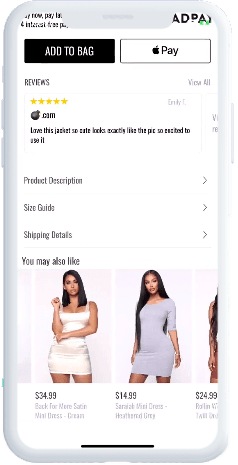This is a detailed screenshot of a mobile phone interface showcasing a shopping page dedicated to women's dresses. The screenshot is framed by a sleek, silvery-gray border mimicking the outline of a modern mobile device. 

At the very top of the interface, there are two prominent action buttons. The first is a black button with bold white text reading "Add to Bag." Adjacent to it, on the right, is a white button with a black outline displaying the Apple Pay logo in black along with the text "Pay."

Directly beneath these buttons is a reviews section. A single review is shown, featuring a five-star rating denoted by gold stars. The user "Cam" has commented, "Love this jacket! So cute, looks exactly like the pic. So excited to see it!"

Following the reviews, there are several expandable information rows. These rows include sections titled "Product Description," "Size Guide," and "Shipping Details," each with a right-facing triangular bracket at the edge, indicating the ability to expand for more information.

Further down the page, a recommendation section titled "You May Also Like" features additional dress options. The first highlighted model is a young female wearing a tight-fitting white skirt, which is short in length, priced at $34.99. The second model, a black female with long hair, sports a tight-fitting light-purple dress that offers more shoulder coverage but is similarly short on the legs, priced at $14.99. A third option, partially visible, is priced at $24.99, showing only part of the model's right arm and some of her hair.